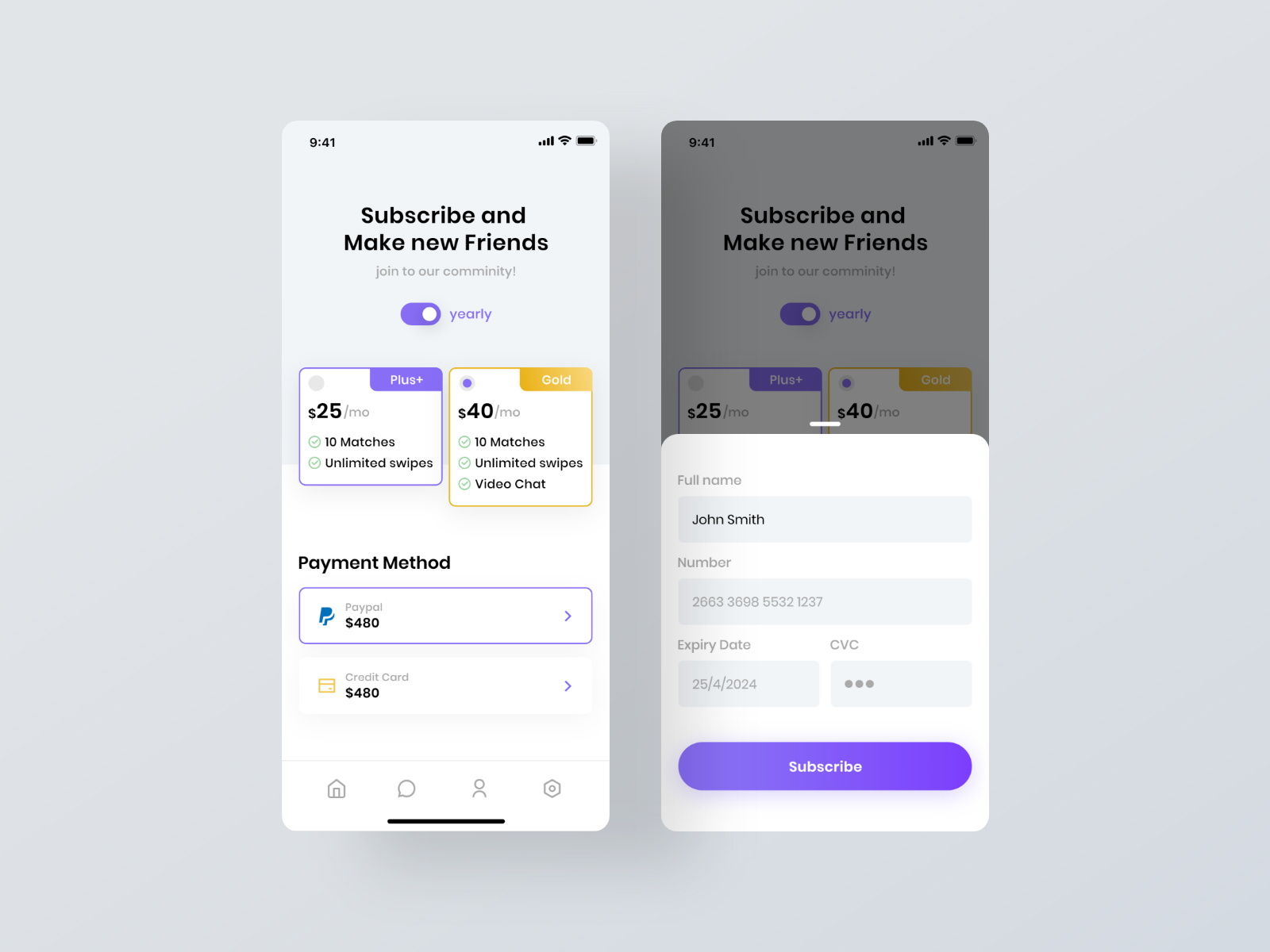The image captures a phone screen displaying two distinct subscription pages for a friend-making app. The first page shows a vibrant, fully powered phone with a strong connection and a time stamp of 9:41. It prominently features the text "Subscribe and Make New Friends" at the top. 

Underneath, various subscription plans are advertised:

- **Yearly Community Plan:** Described with a purple toggle switch that is illuminated, priced at $25 per month. This plan offers 10 matches and unlimited swipes.
- **Gold Membership:** Priced at $40 per month, it provides 10 matches, unlimited swipes, and a video check feature.

The payment methods displayed include PayPal, with a total amount of $480, and an option for credit card which isn't selected. 

The second page, partially visible and grayed out, echoes the "Subscribe and Make New Friends" message. It is overlaid by an active pop-up window requesting user details for payment. The form fields include the user's full name (filled as John Smith), credit card number, expiration date, and CVC number.

At the bottom, a prominent purple bar with rounded edges and the word "Subscribe" invites users to confirm their subscription after correctly entering all necessary information.